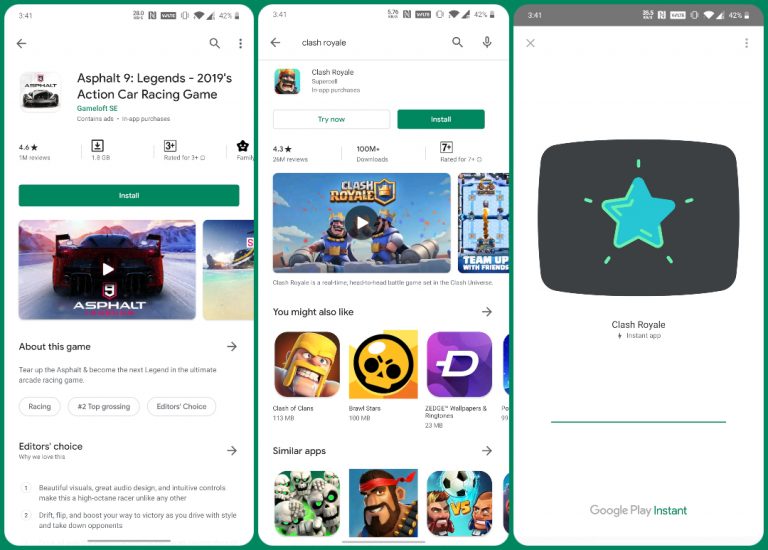Three screenshots captured at 3:41 PM with a battery level of 42%.

1. The first screenshot features the top bar with a left arrow, magnifying glass, and three vertical dots. Below, it showcases the game "Asphalt 9: Legends" with a detailed description. The game is listed as a 2019 action car racing game with a 4.6-star rating based on approximately 1 million reviews. It holds the number two position in top grossing games, as indicated by a "Top" badge with a star. Additionally, it is marked as an "Editor's Choice."

2. The second screenshot displays the game "Clash Royale." The top bar features a left arrow, magnifying glass, and a microphone. The game title "Clash Royale" is shown alongside options to "Try Now" in a green rectangle and "Install." This game has a 4.3-star rating with around 25 million reviews, although the text size makes it difficult to discern between 2 million and 25 million reviews.

The overall layout and visual elements, including the consistent presence of navigation icons and game descriptions, provide a comprehensive view of popular mobile games available at the time of capture.